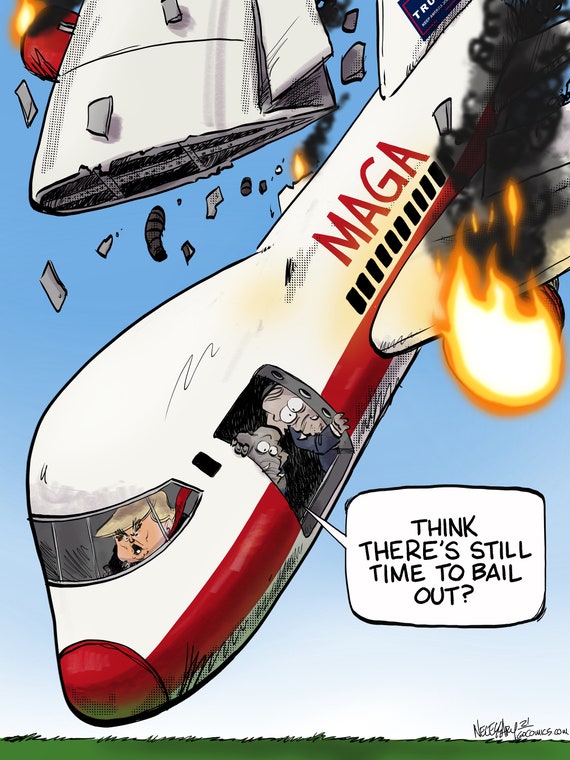This is a vertical, political cartoon depicting a dramatic scene of a white plane with a red stripe, labeled "MAGA" in red font, nose-diving towards the ground. One wing is broken off and floating up, while the other is engulfed in flames, emitting yellow fireball and black smoke. The plane is piloted by a caricature of Donald Trump, who appears frantic, with his tie flapping behind his head. Near an open door of the plane, a dog and an elephant —representing political symbols— are looking out with alarm, and a speech bubble from the elephant reads, "I think there's still time to bail out." The sky transitions from dark blue at the top to nearly white at the horizon, and a thin strip of green grass at the bottom marks the impending crash site. The artist's signature, difficult to decipher, is located in the bottom right corner of the image.